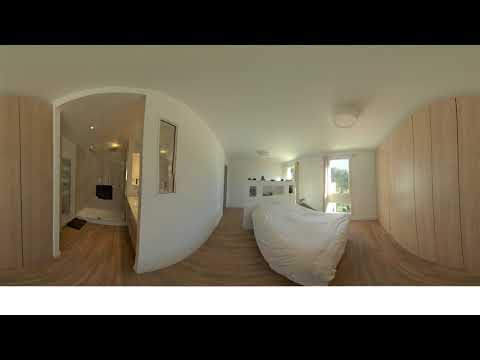This panoramic image, displaying a fisheye-distorted view, captures a detailed interior of a bedroom with an adjoining bathroom. The room features light brown wooden hardwood floors and very light brown walls with a panel-like appearance, while the ceiling remains crisp white adorned with a white light fixture. Positioned centrally is a white bed complete with white sheets and a white headboard. To the right of the bed, there is a tall doorway or window opening onto a balcony, allowing sunlight to filter into the room. On the left, the room extends into the bathroom area, which contains a shower with a tall glass door, a sink, and shelves. A towel hangs on a rack near the sink, and additional lights illuminate this bathroom section. A smoke detector is mounted on the center right ceiling, and no people are present in the room. The photograph appears curved and is bordered with black bars at the top and bottom, with an additional thick white bar overlaying the bottom black bar, suggesting it is a still from a 360-degree image.